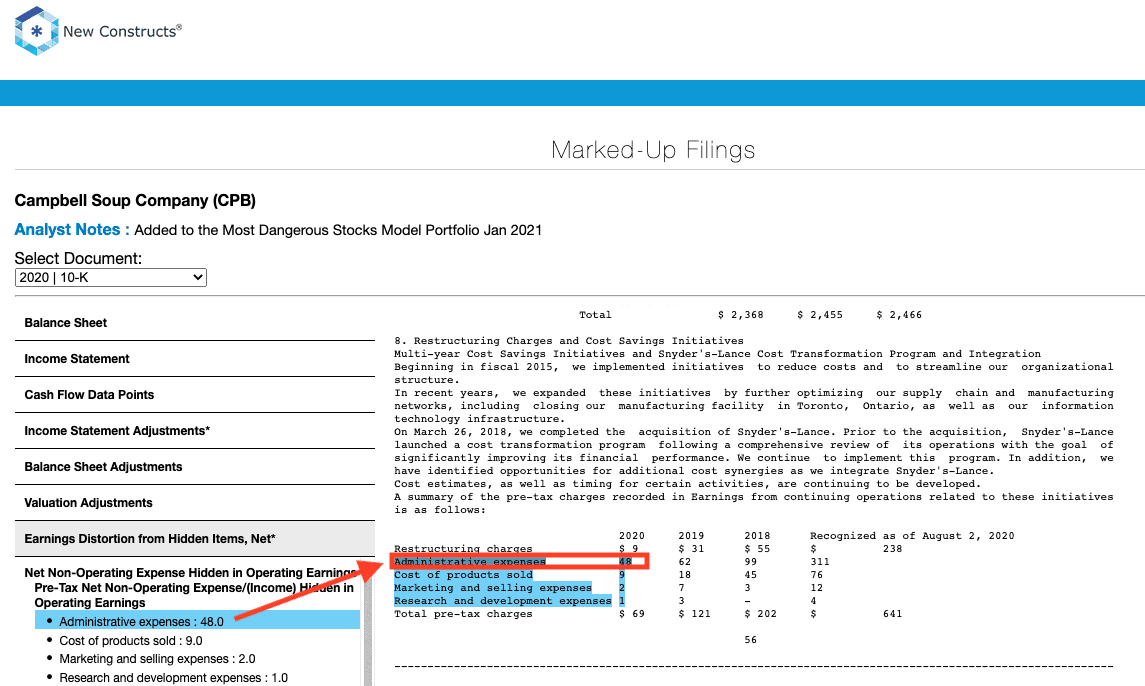Detailed Caption: 

The image is a screenshot from the New Constructs platform, featuring an in-depth financial analysis of the Campbell Soup Company, identified by its ticker symbol, CPB. The analysis highlights that the company's stock was added to the "Most Dangerous Stocks" model portfolio in January 2021. The document selected for review is Campbell's 2020 10-K SEC filing, which provides comprehensive financial data for the fiscal year.

On the left side of the screen, various financial metrics are displayed, including balance sheet items, income statement data, cash flow information, and several types of adjustments such as those for income statement, balance sheet, valuation, and earnings distortions. The middle of the screen shows a detailed view of the income statement, with a specific focus on administrative expenses, which are highlighted and recorded as $48.0 million.

The document mentions extensive text, albeit in very small font, discussing the company’s restructuring charges and cost-saving initiatives. These notes elaborate on multi-year savings efforts aimed at improving financial health and operational efficiency. The highlighted analysis points suggest a meticulous review, indicating significant financial scrutiny on Campbell Soup Company's administrative expenditure and ongoing restructuring programs.